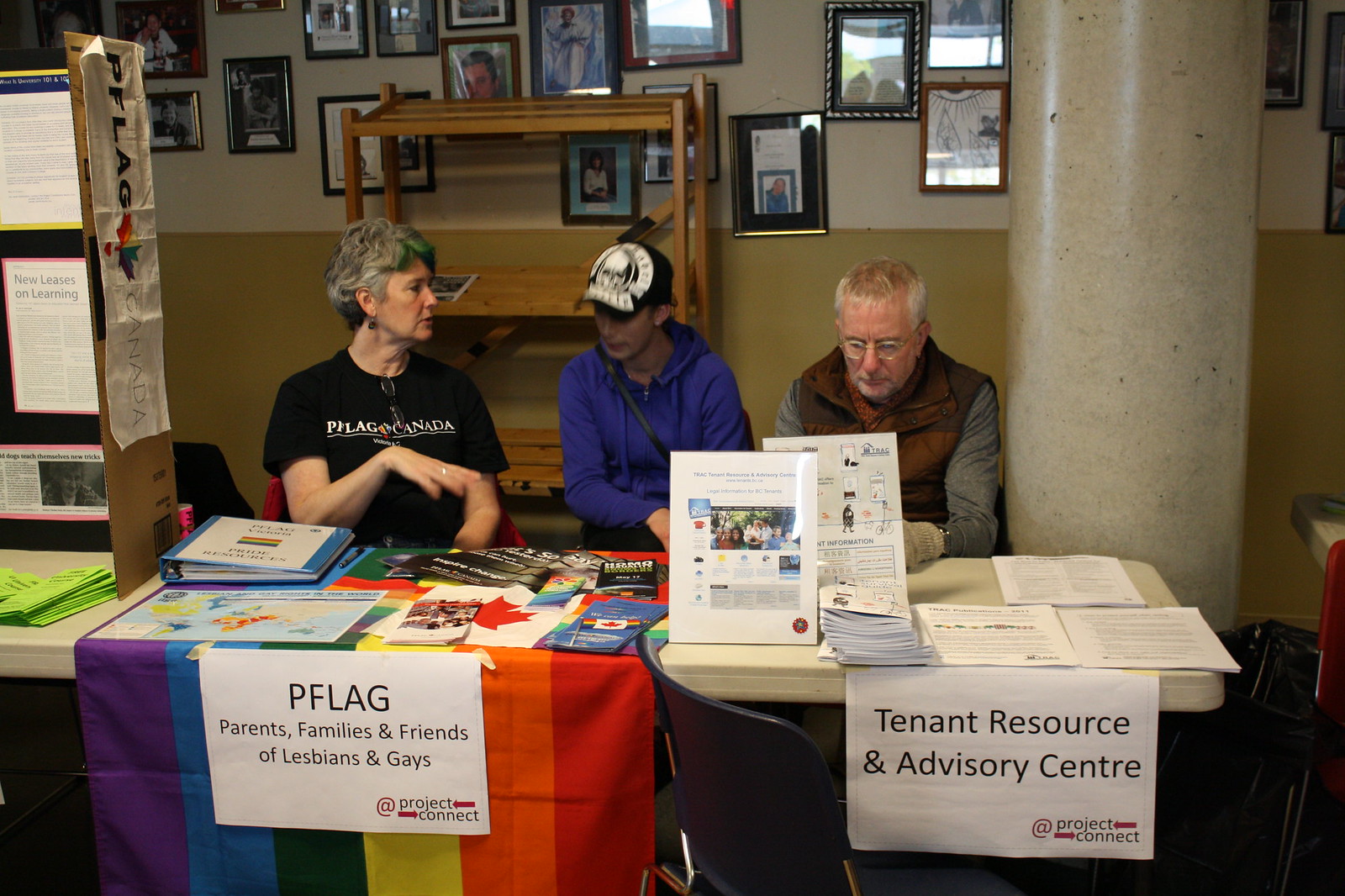In the image, three people are seated behind a long table indoors, likely during the middle of the day at a resource or school event aimed at providing information about different groups. The table, covered with various pieces of literature, booklets, and pamphlets, is split by two signs: on the left is a rainbow flag with a white sign that reads “PFLAG: Parents, Families, Friends of Lesbians and Gays,” and on the right, a smaller sign labeled “Tenant Resource and Advisory Center.” The individuals at the table include a woman on the left in a black t-shirt, looking to her side while speaking with the person in the middle, who sports a black and white baseball cap and a blue hoodie. The third person, a man on the right, wears a brown vest over a gray shirt. Behind them, the room is lined with framed photographs and a wooden bookshelf, complemented by a white pillar. Additionally, on the left side of the image, there appears to be a collage setup with various pages attached, contributing to the informative and resourceful ambiance of the setting.